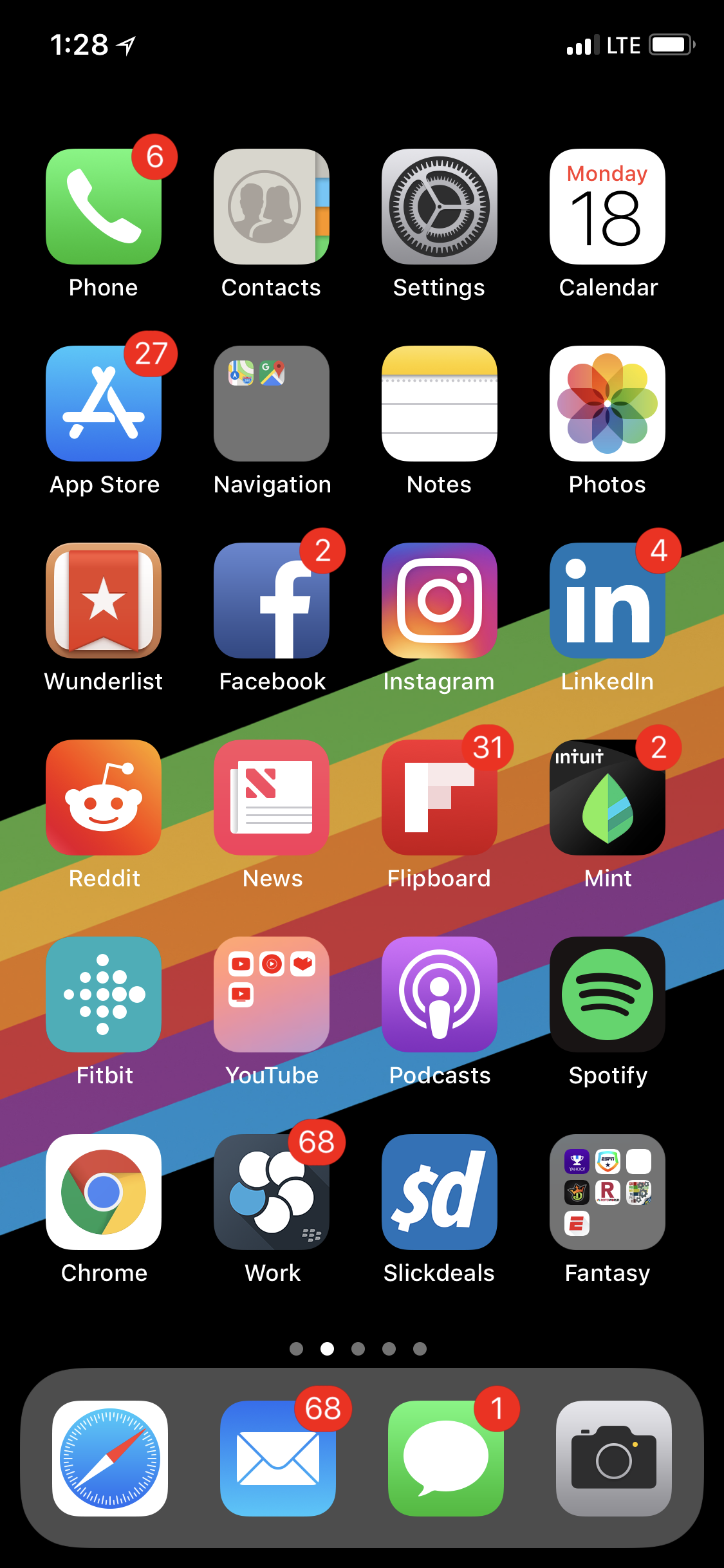A detailed screenshot of an iPhone home screen is depicted. At the very top, the status bar displays "128" with an adjacent pointer icon whose significance is unclear. The status indicators include three bars of signal strength, LTE connectivity, and a mostly full battery. The screen showcases an array of app icons. At the bottom, there is a gray lozenge containing four primary app icons: the Safari browser icon (suggesting this is indeed an iPhone), an email app icon represented by a blue envelope with a red badge indicating 68 unread messages, a green chat bubble with a notification badge of one new message, and a camera icon. Additionally, many more app icons are visible on the screen, including a folder labeled "Fantasy," which contains seven smaller icons within it, hinting at various apps related to that category.